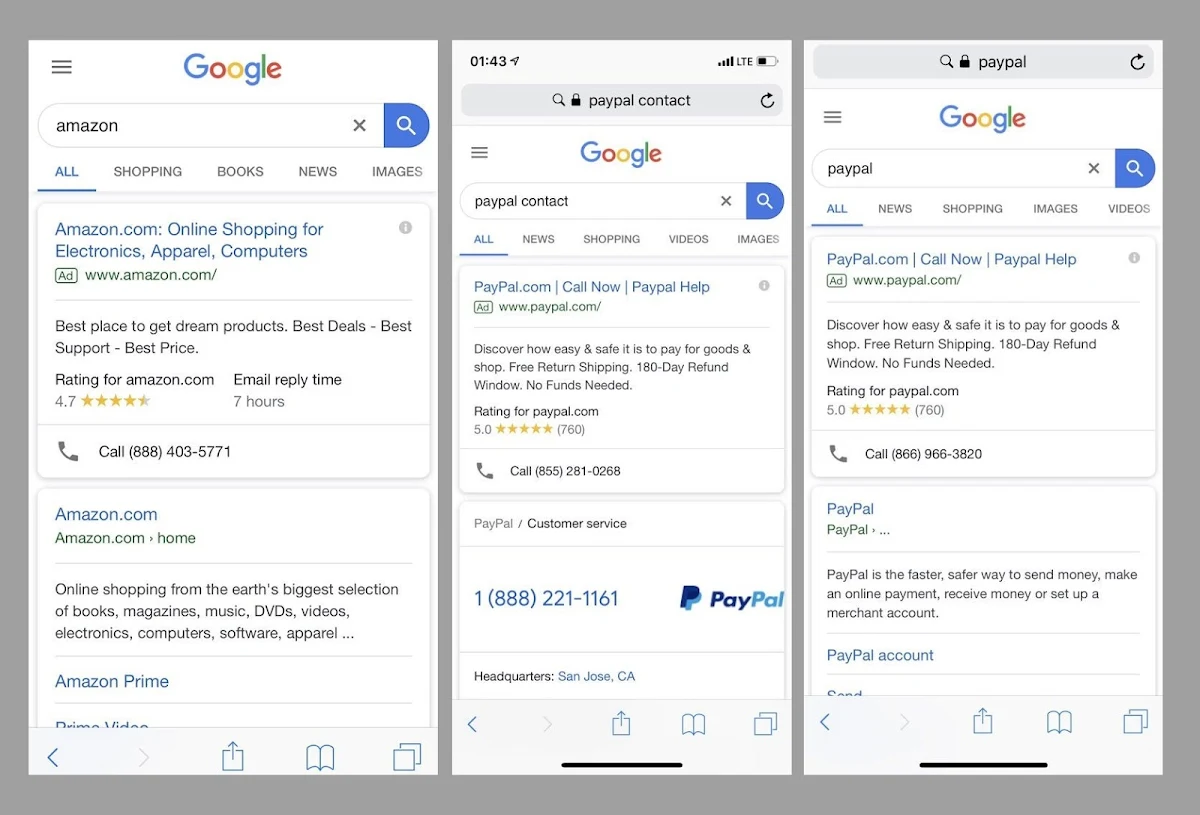This image consists of three separate phone screenshots, each highlighting different Google search result pages. 

The first screenshot displays a Google search in portrait orientation. The Google logo is prominently featured at the top, followed by the search bar where the user has typed "Amazon." Underneath the search bar are various filter buttons: All, Shopping, Books, News, and Images. The top search result is an advertisement for Amazon.com with the tagline "Online shopping for electronics, apparel, computers," accompanied by the website URL (www.amazon.com), a claim about being the best place for dream products, deals, support, and prices, a 4.7-star rating, and a response time for emails listed as seven hours. Following the ad is the first organic search result for amazon.com.

The second screenshot is taken at 1:43 PM, as indicated by the top bar, which also shows a full service bar and a half-full battery icon. This search queries "PayPal contact" in Google. The first result is an advertisement for PayPal, and the highlighted answer is the PayPal customer service phone number: 1-888-221-1161.

The third screenshot, similar to the second search, shows another Google search results page for "PayPal." The advertised result for PayPal appears at the top, followed by the first non-advertised link for PayPal.com.

Each screenshot provides essential search information, clearly illustrating the user's intent to find contact details and websites for well-known services like Amazon and PayPal.